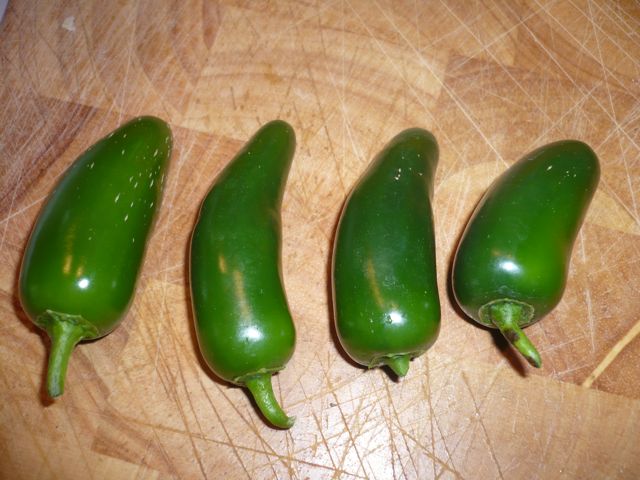This up-close photograph captures four jalapeno peppers, arranged in a row, on a light brown wooden cutting board. Each jalapeno has a bright green stem, contrasting with their darker green, shiny bodies that reflect the camera's flash at the bottom. The peppers vary slightly in size and shape: some are a bit fatter or shorter, but they all share a similar curved orientation with their stems pointing down. The cutting board, heavily worn from extensive use, displays a multitude of knife gouges in various directions, adding rich texture and evidence of its long history in the kitchen. No text accompanies the image, which centers perfectly on the peppers, emphasizing their uniform yet individual appeal against the rustic backdrop of the well-used cutting board.